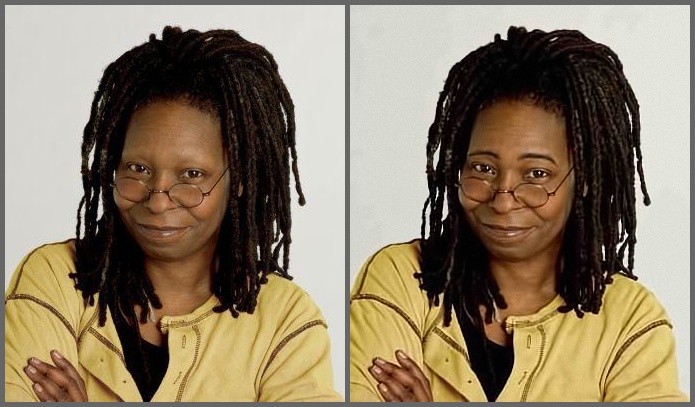The image depicts actress and talk show host Whoopi Goldberg in a professional photograph set against a white or gray background. There are two side-by-side pictures of her, both showing her with her signature brown dreads, round glasses perched at the end of her nose, and a subtle, Mona Lisa-like smile. She is dressed identically in a yellow shirt layered over a black shirt, with her arms folded. The primary distinction between the two images lies in her eyebrows: the left image shows her without discernible eyebrows, while the right image appears to have digitally added, darker eyebrows. This subtle alteration highlights the contrast while maintaining her overall look and expression.